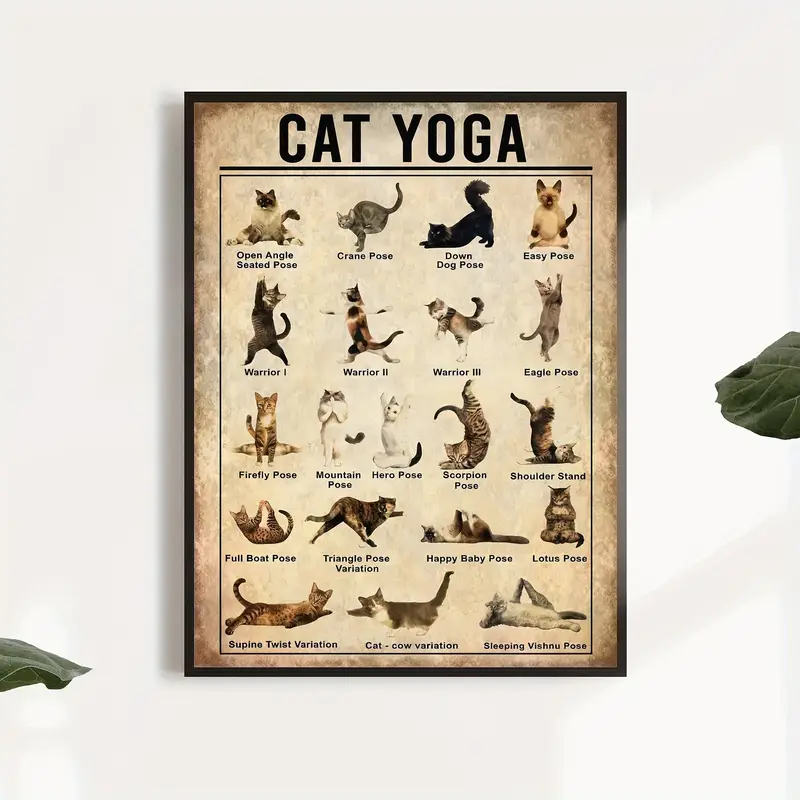The photograph depicts an artwork titled "Cat Yoga," prominently displayed on a solid white wall. The piece is framed with a thin, dark-brown frame and features a poster of a brownish-beige hue. At the top, the title "Cat Yoga" is inscribed in bold black letters, accompanied by a long cat illustration. The artwork consists of roughly 20 individual illustrations of cats, each performing a different yoga pose. These positions range from Open Angle Seated Pose and Downward Dog to Crane Pose, Eagle Pose, Warrior Poses, Firefly Pose, Easy Pose, Happy Baby Pose, and Scorpion Pose, among others. Each cat is meticulously drawn to mirror traditional yoga postures, with every illustration clearly labeled. Surrounding the central artwork, parts of green leaves are visible on either side, contributing to the overall aesthetic.